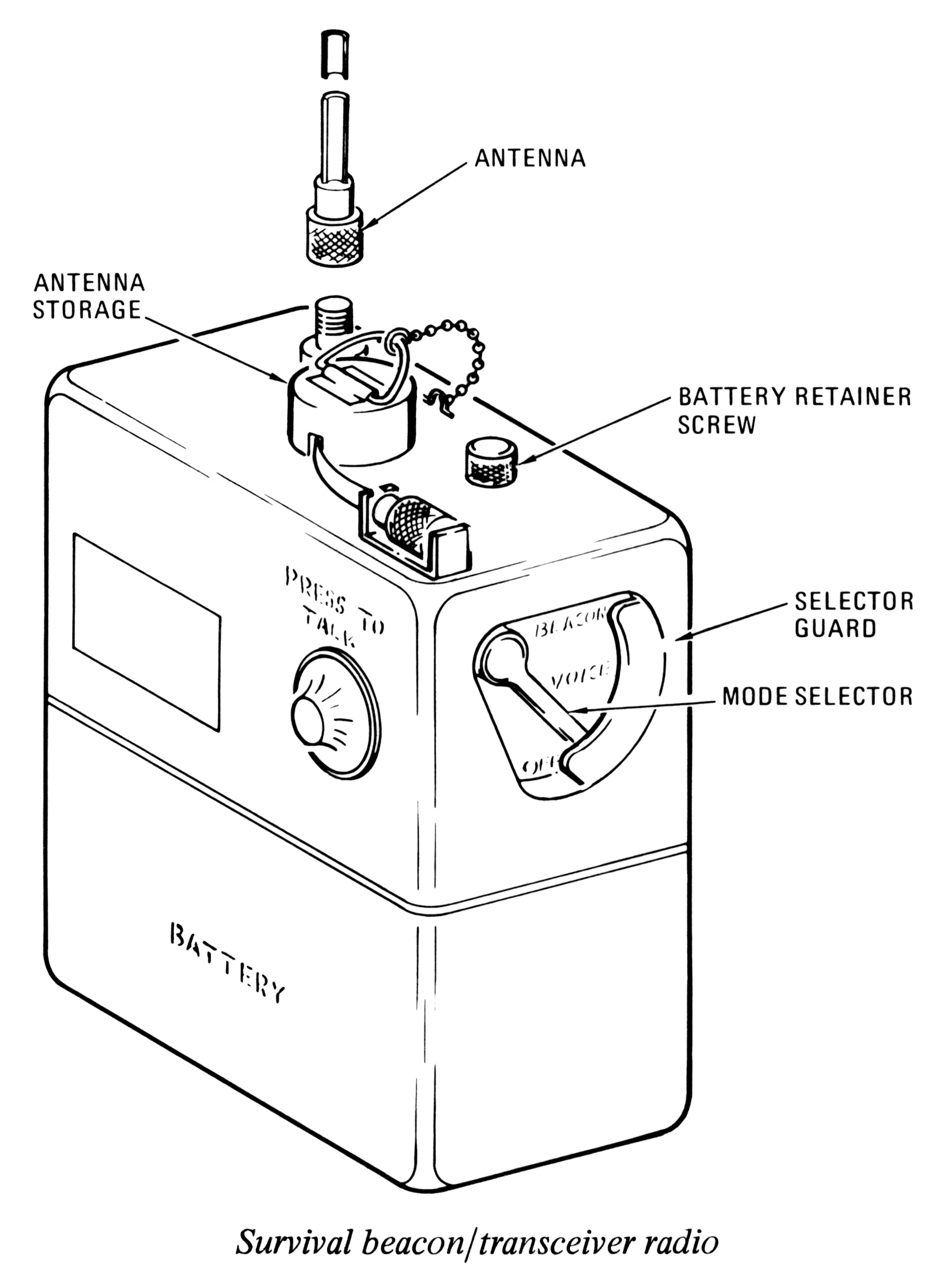This black and white diagram depicts a survival beacon transceiver radio, prominently labeled at the bottom of the illustration. The drawing, rendered in simple pen strokes on a plain white background, meticulously identifies each component of the device. At the top, the antenna is shown detached for clarity, alongside its corresponding storage unit, which features a cap secured with a chain. The illustration also highlights two bolts near the antenna storage area.

Central to the design is the mode selector, which allows the device to switch between various modes, safeguarded by a selector guard to prevent accidental changes. A "press to talk" button is prominently displayed, indicating the radio's walkie-talkie functionality. Further details include a battery retainer screw and a small screen that likely displays essential information. Located at the bottom of the device is the battery compartment, crucial for powering the unit. This compact and efficient layout suggests the radio is designed for emergency scenarios, emphasizing practical usability and straightforward access to its features.